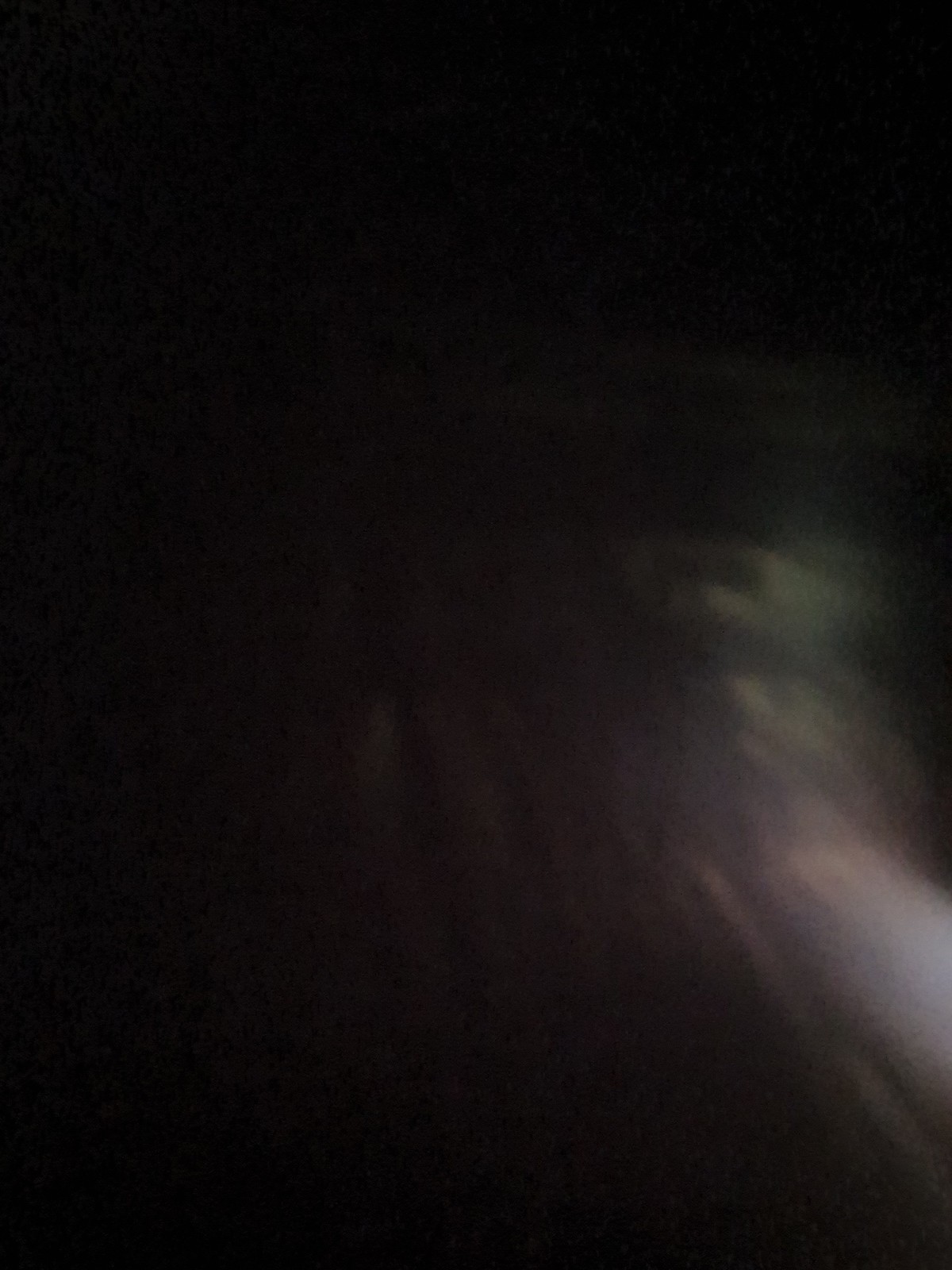This vertical photograph is minimalist in nature, with the frame predominantly filled by an expanse of near-total darkness. The deep, inky blackness lacks discernible details, creating a stark and mysterious canvas. In the bottom right corner, however, a faint, ghostly haze introduces a subtle hint of color and texture to the composition. This haze, rendered in delicate shades of grayish-purple with occasional hints of green, suggests a slight motion blur, indicative of an image taken in low light conditions. The camera's slow shutter speed has captured the ethereal, indistinct blur of something illuminated, adding an element of dynamic movement. Upon closer inspection, the hazy area reveals fine grain and texture within its amorphous shape, though its exact nature remains elusive, evoking a sense of enigmatic beauty amid the surrounding darkness.